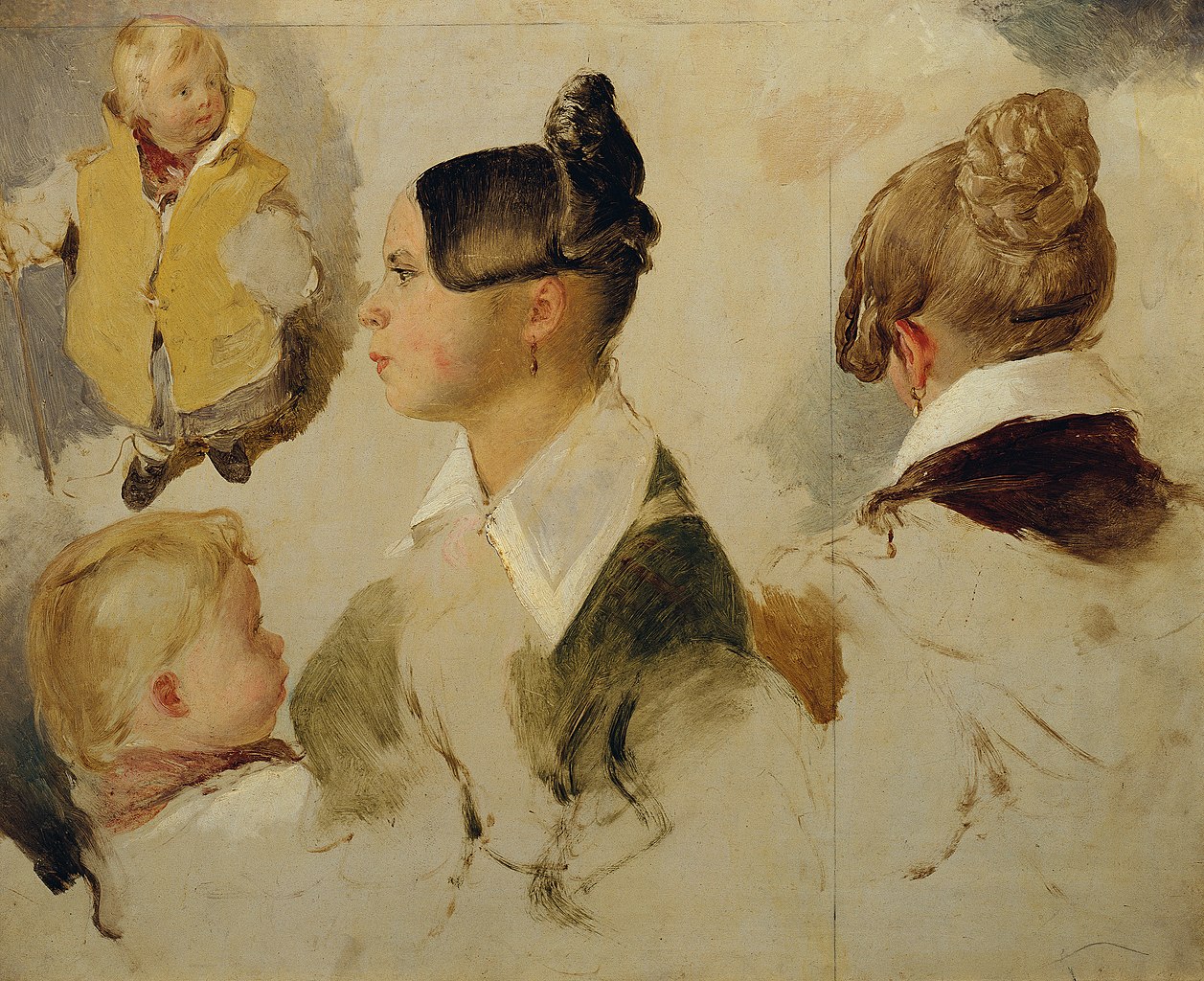The image is a detailed portrait featuring four individuals rendered in a sketch-like style. Central to the composition is a mid-30s to 40s woman with blonde hair styled in a bun, visible from a profile view, adorned with a large collar and a dangling earring. She is gazing to the left of the image. Just in front of her and looking over her right shoulder is a small blonde-haired child with chubby cheeks, who appears to be observing another figure. In the background to the right, there is another adult woman depicted from behind, with her blonde hair also styled in a bun, and she is looking away from the viewer. On the upper left side of the composition, a second child, also blonde and dressed in a brown parka coat with the collar pulled up, is standing and looking into the upper right corner of the image. The overall scene is bathed in a brownish, bleached-out tone, contributing to the sketch-like and nostalgic atmosphere of the portrait.